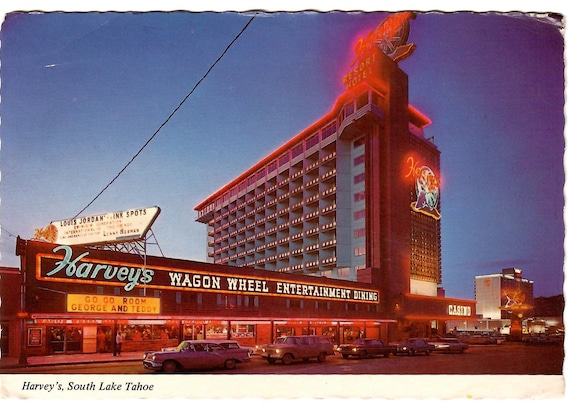This retro photograph, with its fringed edges and a caption at the bottom reading "Harvey's, South Lake Tahoe," depicts an old casino-hotel scene likely from the 1970s. The photograph captures a sprawling, flat three-story building extending almost an entire block, marked prominently by a sign that reads "Harvey's Wagon Wheel Entertainment Dining" in large, illuminated letters. Adjacent to this structure on the right is a significantly taller hotel tower, about nine floors high, each adorned with bright red lights. Below the main sign, a yellow banner advertises "Go-Go Room George and Teddy." The sky overhead is a clear blue, complementing the vivid orange hue of the casino exterior. The image also features classic cars from the 1950s, 60s, and 70s, enhancing the nostalgic feel of the scene, reminiscent of old Vegas.